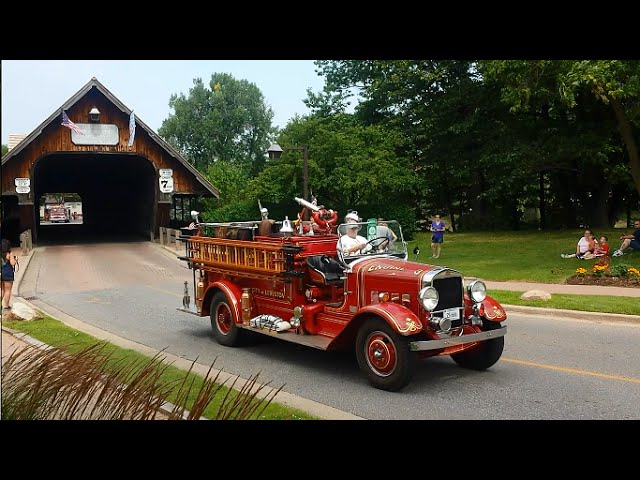This photograph captures an antique red fire truck, adorned with yellow trim and a silver bell, driving on a road. The fire truck, likely restored for parades, has an open, convertible-like design with the driver dressed in a white shirt and hat. To the left, a historic wooden covered bridge displays the number 7, an American flag, and a bell at its roof. Through the dark tunnel of the bridge, another fire truck can be seen approaching. The foreground and background are rich with dark green foliage. On both sides of the road, people are seated on the grass, suggesting a parade-like atmosphere. The right side of the photograph features a garden with yellow and green flowers, where more spectators are gathered, enhancing the scene's lively and festive ambiance.